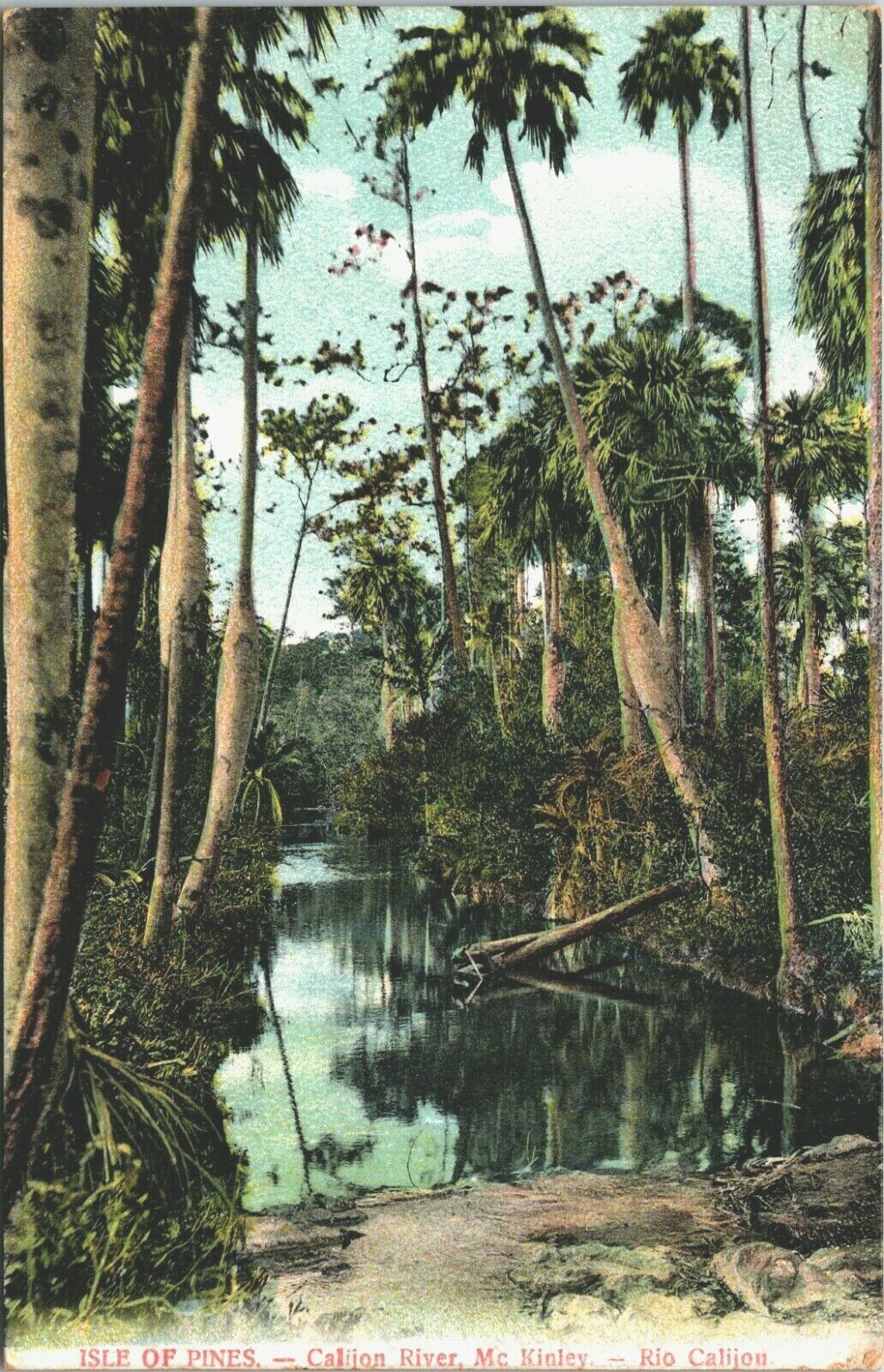The image, a vintage color postcard titled "Isle of Pines, Calajon River, McKinley, Rio," captures a serene tropical scene featuring tall, slender palm trees with leaves crowning their tops. These majestic trees are surrounded by lush green vegetation typical of a tropical setting, devoid of any flowers or bright colors. The scene takes place at the foot of a small river or stream, where the still water reflects the tall palms and scattered clouds in the blue sky above. Fallen tree trunks stretch half onto the land and half into the water, adding to the tranquil and untouched nature of the landscape. Sandy land juts into the water, suggesting a potential boat launch area. In the distance, cliffs or mountains rise, enhancing the setting's peaceful and secluded atmosphere. The colors in the postcard are muted and dull, characteristic of its vintage quality. No human presence disrupts the calm of this picturesque, sunlit day, making it a quiet, serene escape into nature.